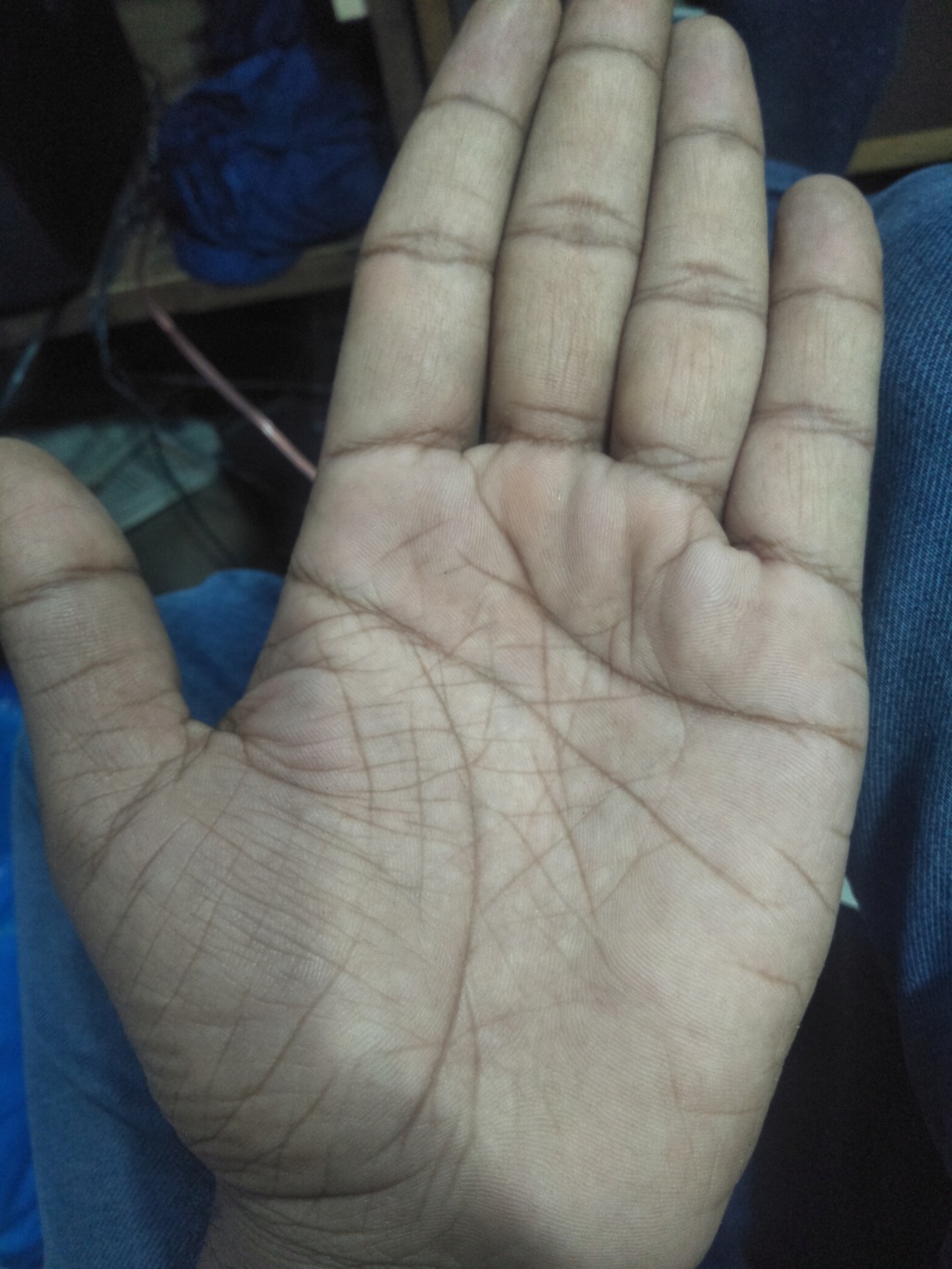In this detailed image, the focus is on the left palm of an individual with brown skin, heavily lined and seemingly belonging to an older male, possibly in his 60s or 70s. The hand appears slightly dirty and is placed palm-up, front and center of the photograph. The thumb is extended, and the other four fingers are held together, showcasing distinct lines along the palm and fingers. The individual is wearing blue jeans, and their palm is resting on their leg. The backdrop includes a cluttered bedroom scene with a blue shirt or blanket bundled up, electronic devices, and power cords scattered across a dark gray floor. Additionally, wooden shelving divided by wooden beams into cubbies holds more blue clothing items.